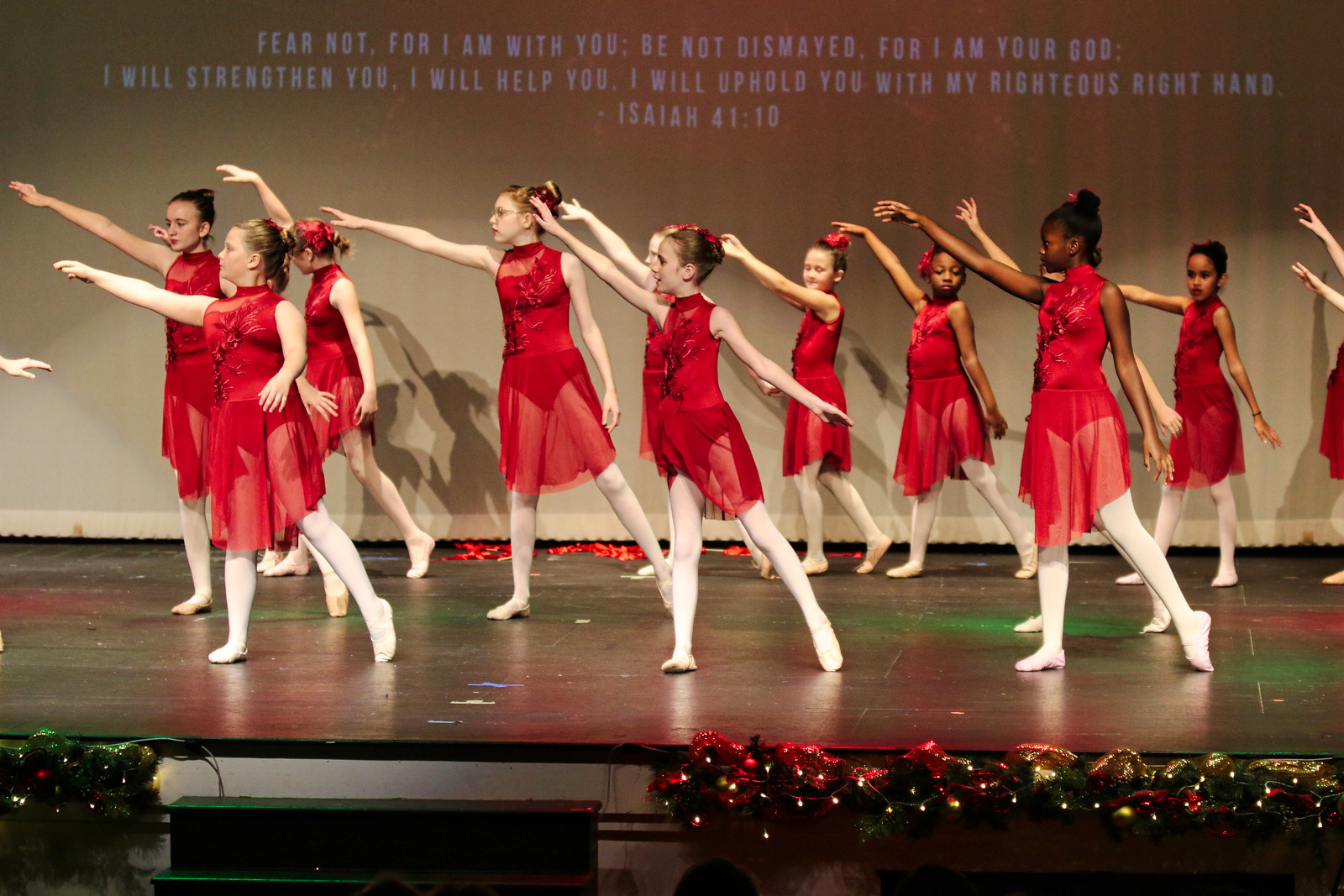The image showcases a girls' dance troupe performing on stage, presumably during a Christmas event at a church. The young dancers are captured in a unified pose, extending their right hands to their sides while balancing with their other arms. They are adorned in red, knee-length dresses with lacy elements and white leggings, complemented by white ballet slippers. The girls' hair is uniformly tied back, and some wear glasses and lipstick. The group includes a diverse mix of ethnicities, with two black girls on the right.

The stage is festooned with festive decorations, including Christmas wreaths adorned with lights and gold ribbons positioned at the bottom of the stage. The flooring appears to be hardwood, with strings of miniature lights and a wiring outline visible along the stage’s edge. In the background, a white scrim displays a Bible verse: "Fear not, for I am with you. Be not dismayed, for I am your God. I will strengthen you, I will help you, I will uphold you with my righteous right hand" from Isaiah 41:10. The text appears in bluish-white letters against the brownish backdrop. The red and green stage lighting further accentuates the holiday ambiance.